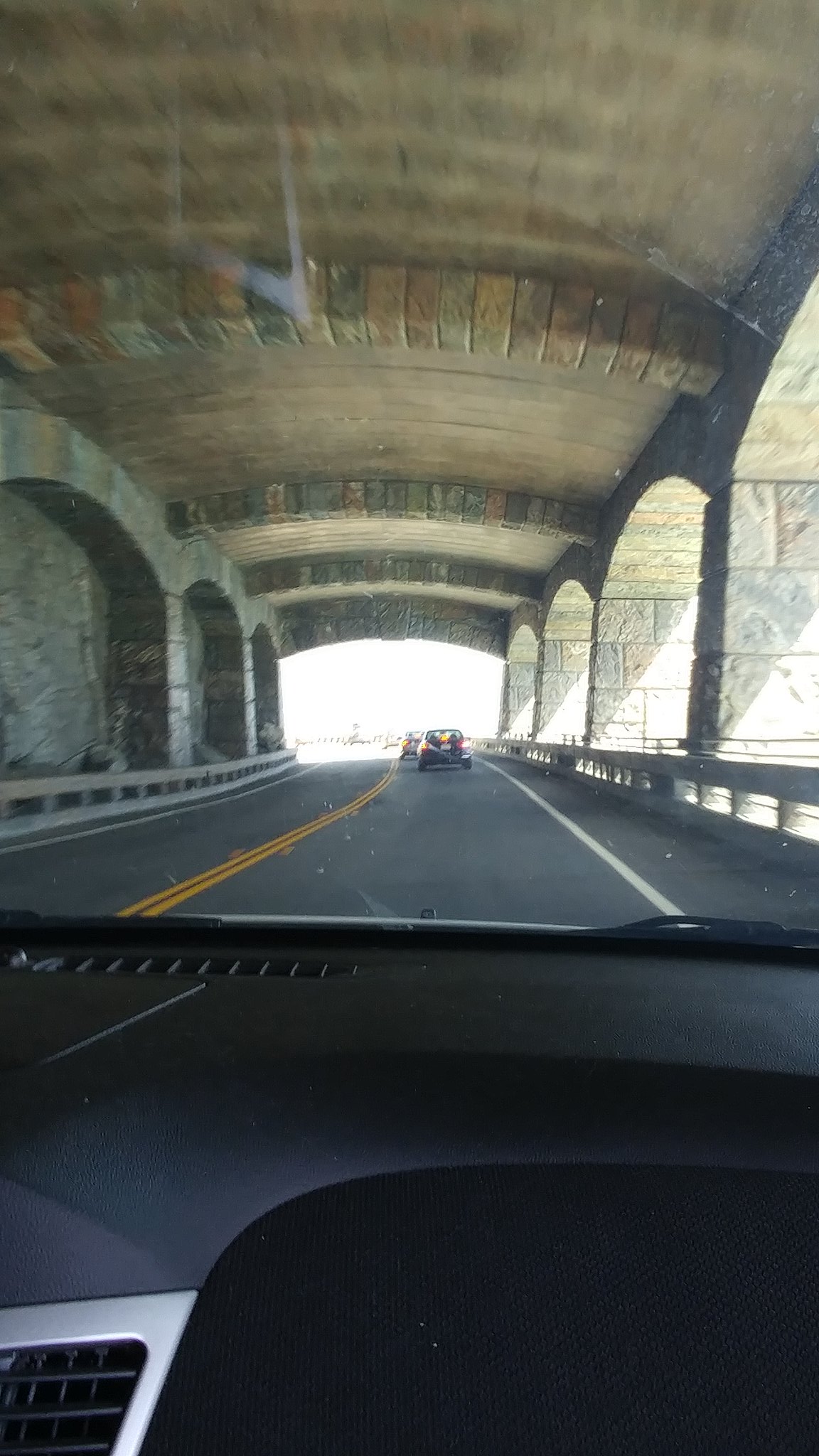This photograph was taken from the perspective of a car driving on a black asphalt road, with the viewpoint through the vehicle's windshield. The car is traveling in the right lane, marked by a solid white line on the far right and a double yellow line to the left, indicating no passing. Guardrails made of gray and silver metal run along both sides of the road, providing a protective barrier.

The road goes under a stone bridge, showcasing its intricate architecture. The bridge features a ceiling made of brown stone with horizontal rows of colored stones resembling beams that add texture and contrast. On the right side of the bridge, there are arches through which sunlight filters, illuminating parts of the roadway. Similar arches are present on the left side, but instead of open views, they reveal a solid stone wall.

In the lower part of the photograph, the top section of the black dashboard is visible, framing the scene from inside the car. At the far end of the image, bright white light signifies the exit of the underpass, suggesting the car's movement toward emerging from beneath the bridge.